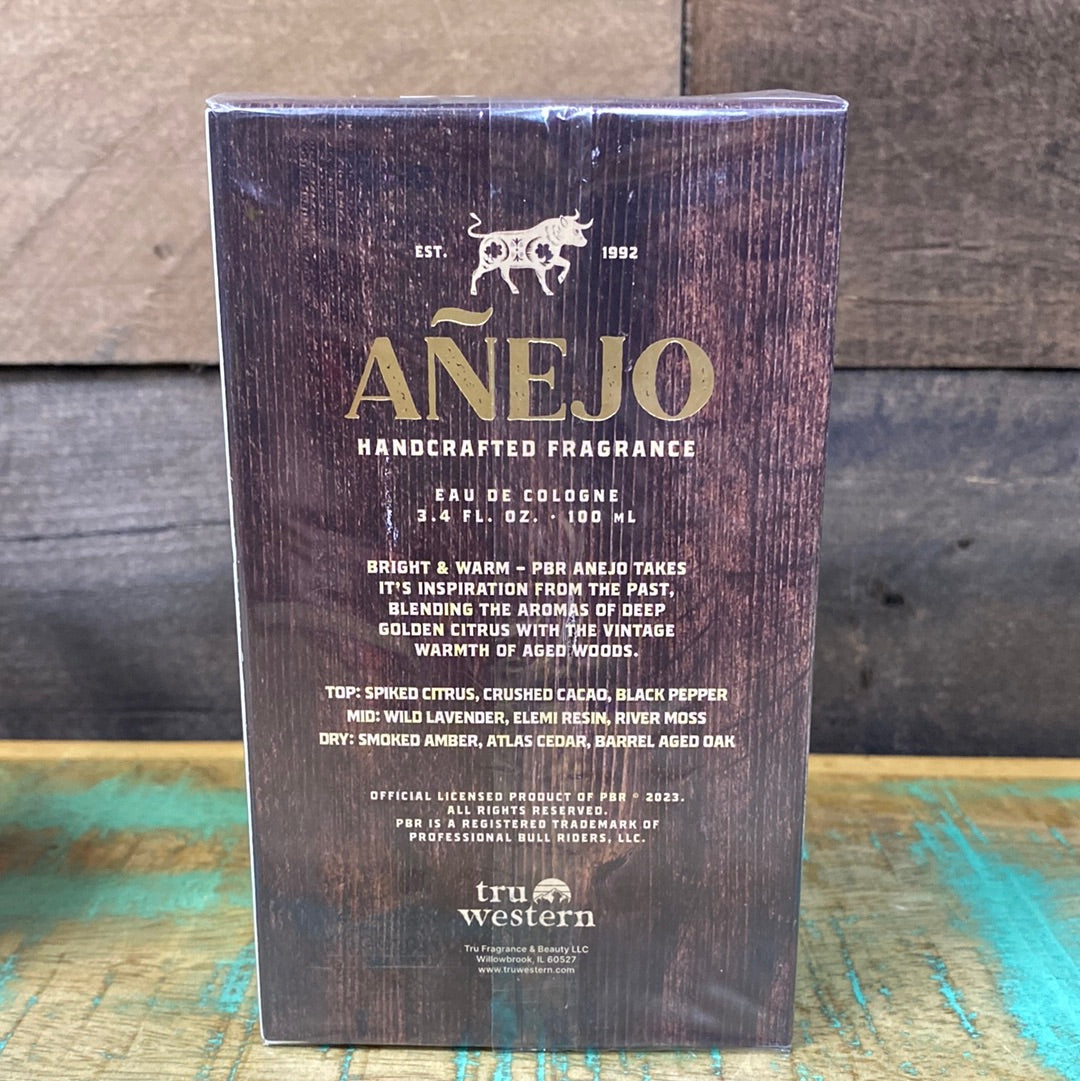This image features a brown, rectangular package of handcrafted fragrance, specifically Eau de Cologne. The package, wrapped in transparent plastic and sealed with tape, is set on a blue-white-yellow-grayish wooden surface with a rustic wood-paneled wall in the background. The front of the box is adorned with a cream-colored image of a bull and the text "EST. 1992" printed above the prominently displayed name "AÑEJO" written in gold letters with a tilde over the 'N'. Below, descriptions in cream-colored font specify: "Handcrafted Fragrance, Eau de Cologne, 3.4 fluid ounces, 100 milliliters, bright and warm." It describes the fragrance as taking inspiration from the past, blending deep golden citrus aromas with vintage-aged wood warmth. The fragrance notes are detailed as follows: "Top: Spiked Citrus, Crushed Cacao, Black Pepper; Mid: Wild Lavender, Elimi Resin, River Moss; Dry: Smoked Amber, Atlas Cedar, Barrel-Aged Oak." The box also bears small prints stating it is an official licensed product of PBR and mentions "True Western" at the bottom, indicating its authentic craftsmanship. Additionally, there is a fine-print section detailing "True Fragrance and Beauty LLC, Willowbrook, Illinois."